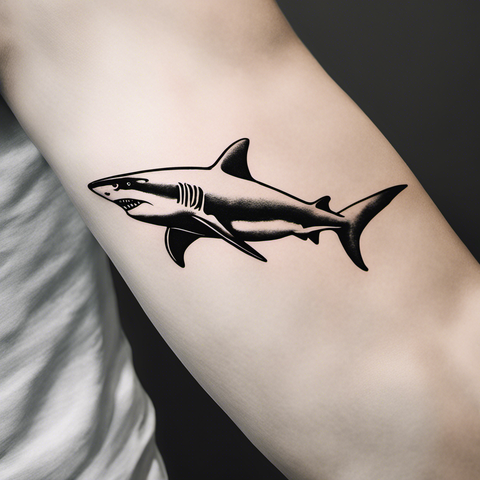The image depicts a pale-skinned person's arm, specifically the inner bicep area right above the elbow. The arm emerges from the upper left corner of the image and extends down to the lower right corner. The person is wearing what appears to be a white tank top, visible in the lower left portion of the image. The background is entirely black, giving a stark contrast to both the arm and the graphic on it.

The focal point of the image is a black and white illustration of a great white shark, positioned as though the shark is swimming in one direction. The shark's head is angled inward toward the person's body, with its tail extending outward. The illustration shows intricate details such as the shark's nose, eyes, teeth, and fins, giving it an intense and sleek look. The graphic appears too clean and polished to be a real tattoo, suggesting it is likely a digital rendition, possibly created through a tattoo app or photoshopped onto the arm to visualize what the tattoo would look like in reality.